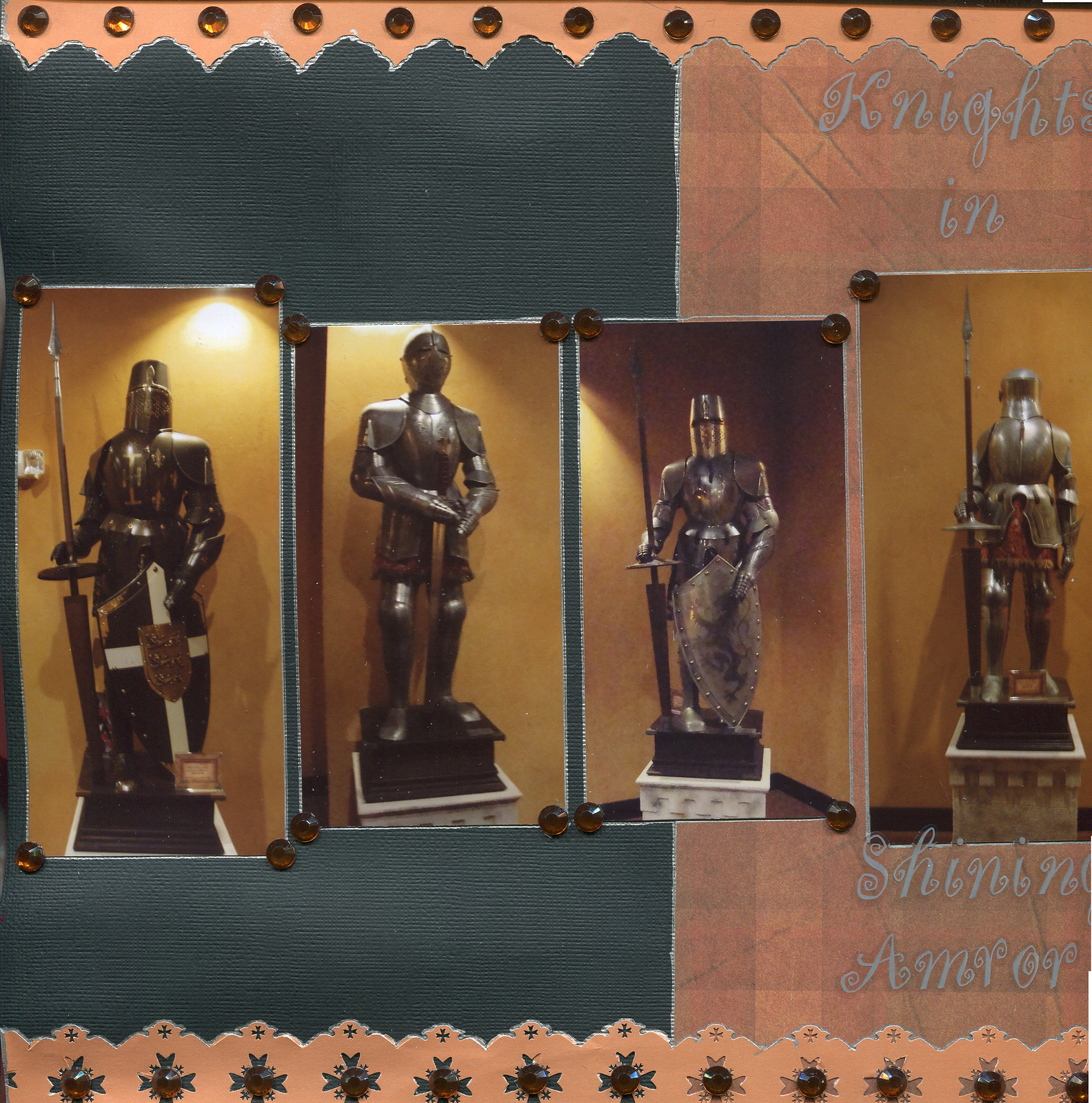This image features a detailed poster-style display showcasing a series of photographs centered around knights in shining armor. The overall background is characterized by an orange hue split diagonally, with one side in a dark green and the other in a tannish orange. The top and bottom borders are adorned with small brown jewels. Prominently, the phrase "Knight in Shining Armor" is written in gray font across the image.

Four distinct photographs are pinned to this split background using the same small, brown jewel accents. Each photograph features a well-preserved piece of knight's armor from various museums, all highlighted against a consistent yellow backdrop.

The first photograph displays a knight with a spear and shield, distinguished by a more bucket-style helmet. The second features a knight with a sword and a closed-mask helmet. The third photograph showcases armor with a coat of arms decorated with a griffin, accompanied by a lance-style weapon. The final image presents a simpler, less decorative suit of armor holding a spear.

This rich and textured backdrop alternates between dark blue on the left-hand side and pink on the right-hand side, enhancing the medieval theme of the displayed armor.